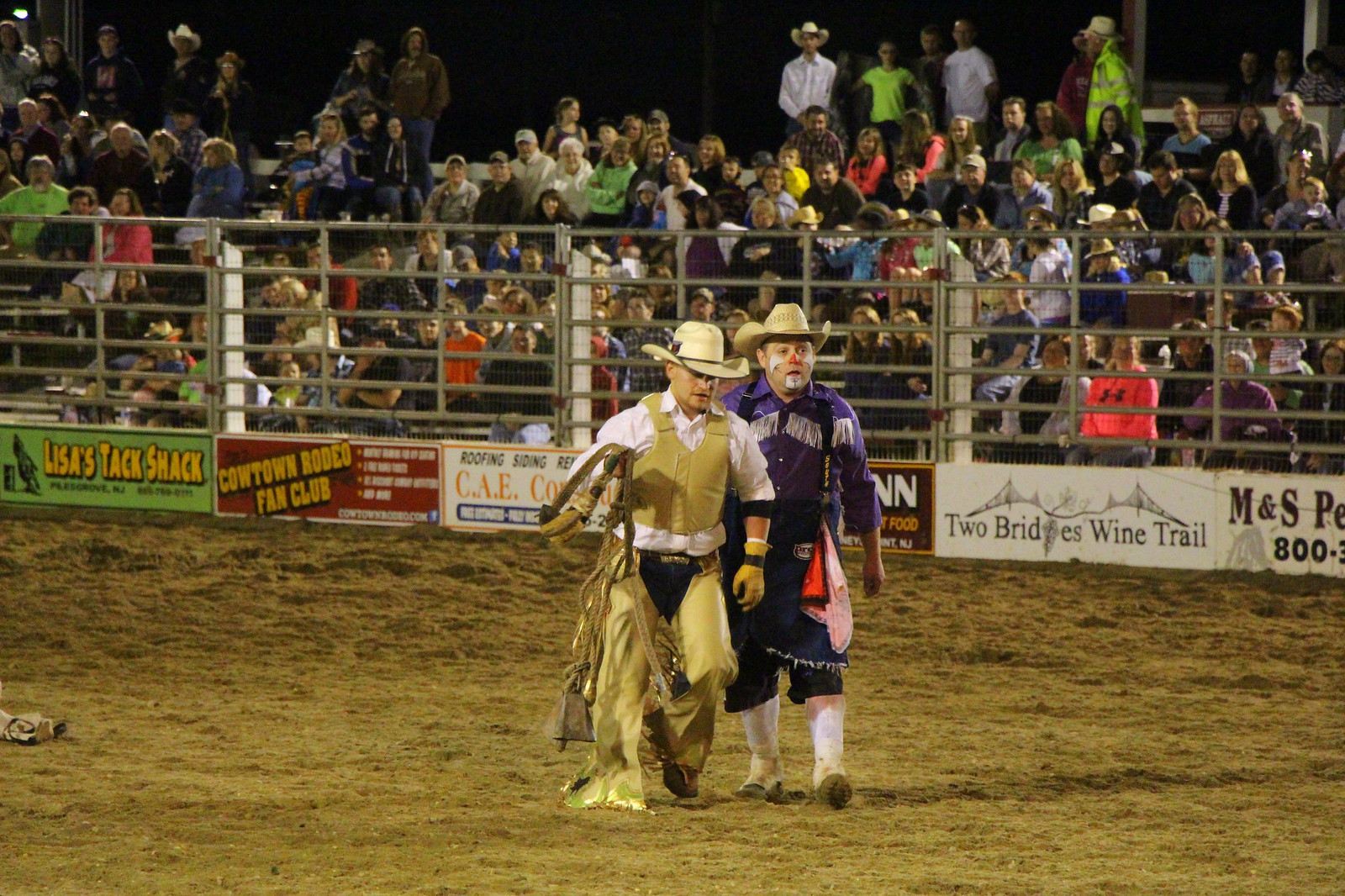In this lively rodeo scene, a central cowboy, dressed in gold-yellow chaps and a matching yellow vest over a white shirt, strides confidently across the barren rodeo surface holding his saddle in his right hand and a glove in his left. His cream-colored cowboy hat adds to his traditional rodeo look. Walking beside him is a flamboyant rodeo clown, distinguishable by his big red nose and face paint. The clown sports a purple fringed jacket and matching trousers, complemented by white socks and shoes, as he follows the cowboy. Both are moving from left to right across the image.

The background showcases the bustling stands packed with a diverse crowd of spectators. From the front row, lined with advertisements like Lisa's Tac Shop in green, Cowtown Rodeo Fan Club in red with yellow lettering, a white sign with orange letters for CAA Roofing Siding, and Two Bridges Wine Trail with a skyline on a white sign with black printing, the fence and the stands are visible. Although some sections have a few empty seats, the overall impression is of a well-attended event with fans of all ages, many wearing colorful shirts and cowboy hats.

Amidst this vibrant scene, the metallic fencing and the varied advertisements serve as a protective barrier while adding a flamboyant backdrop to the cowboy and clown's journey across the rodeo arena. The muddy, grassy foreground transitions smoothly into the central focus, emphasizing the action and excitement of this rodeo event.